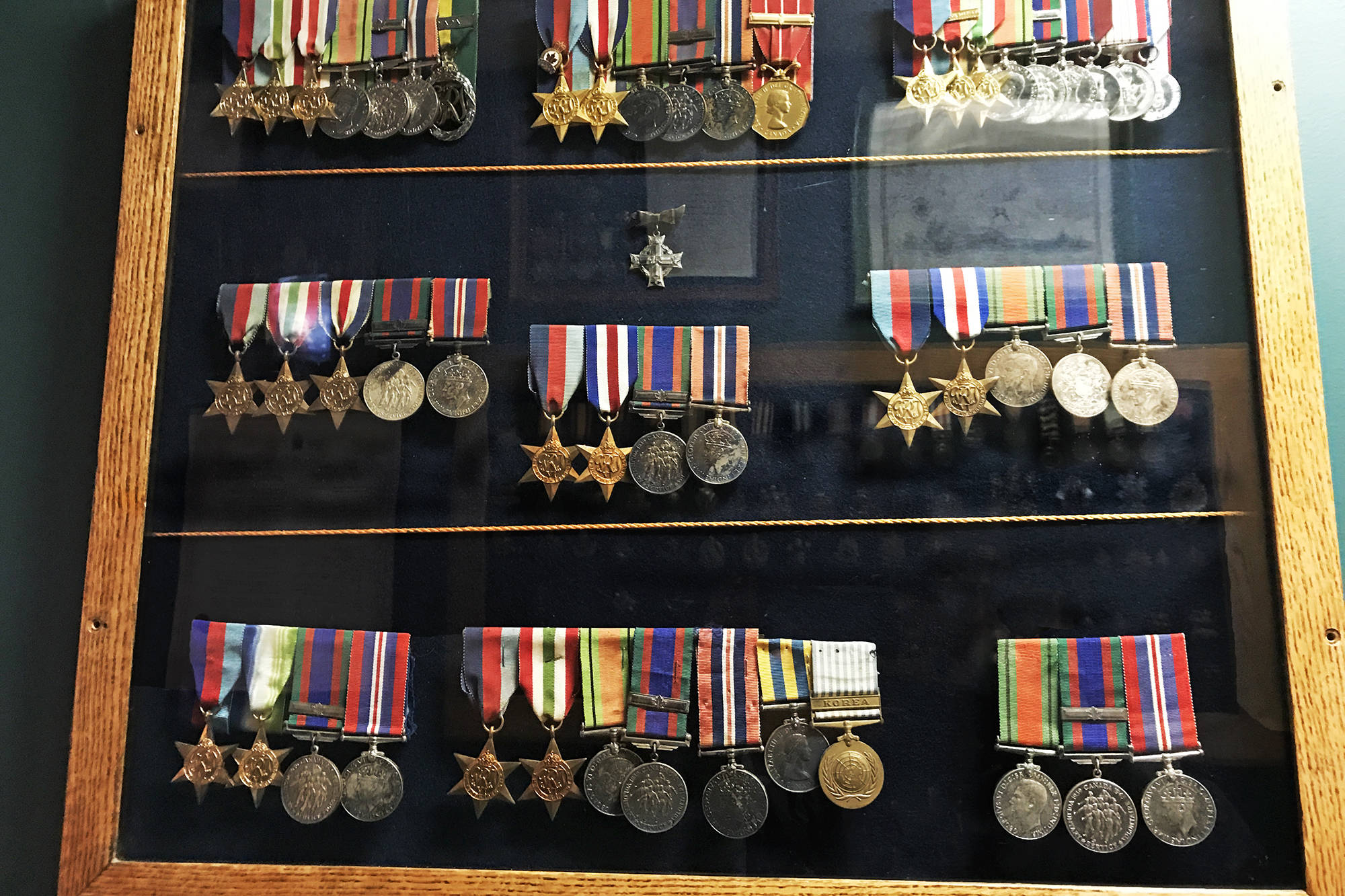The image showcases a large, rectangular shadow box with a wooden frame and a black or navy blue fabric background. The shadow box is wall-mounted and features a glass front, which reflects images from the opposite side of the room. Inside the box, the display is divided into three distinct sections by pieces of twine. Each of these sections contains rows of brightly colored, striped ribbons, each adorned with various medallions. There are three rows in total, with the top row slightly cut off and the bottom row fully visible within the frame.

Each row consists of a collection of approximately 15 military medals, exhibiting a variety of shapes, including round, star-shaped with six points, and cross-shaped. The ribbons are vibrantly striped with colors, such as red with blue stripes and green with an orange stripe. The medallions themselves range in materials and appearances, some being silver or gray, others copper-looking, and some appearing weathered and darker. This intricate display captures an array of old, possibly antique, military awards, highlighting a rich history through their preserved presentation.